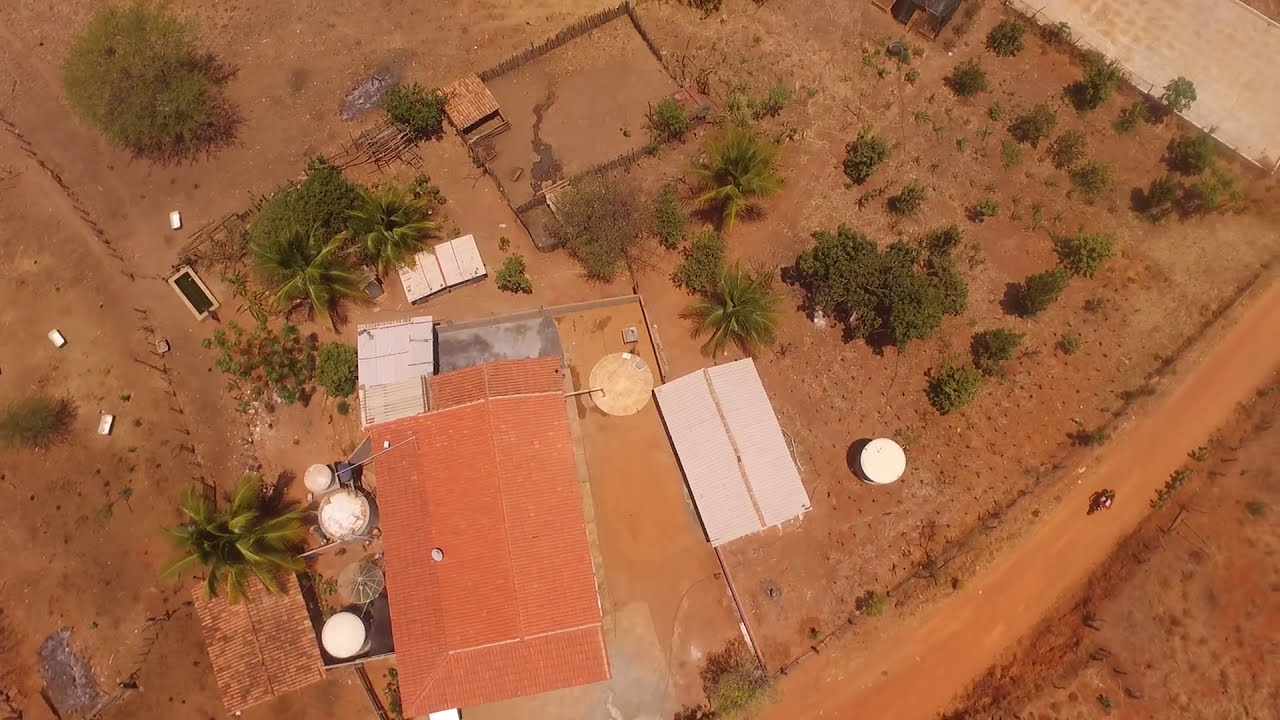The aerial photograph captures a sprawling homestead or farmland set in a dry, desert-like area. At the center of the image is a large building with a distinctive orangish-reddish clay-tiled roof, tapered from the center toward both sides. On the left side of this roof near the bottom, there’s a small gray dot and further down are two silver-colored cylinders, one of which has brown stains. Flanking this large building are various smaller structures, including one with a light silver roof accented by a prominent brown stripe.

Adjacent to these structures is a light brown dirt road running alongside the property, veering from the bottom center to the top right. Travelling along this road is an indistinct vehicle, possibly a motorcycle or scooter. Scattered throughout the property are several palm trees and a variety of other green foliage, but the predominant ground cover is light brown dirt, indicative of a dry climate.

Just above the large building is a corral encircled by a wooden stick fence, which likely serves as a livestock enclosure. Within the corral, there is a smaller structure with an orange and brown roof providing shelter, and a meandering stream of water can be seen crossing the area. The overall scene suggests a secluded, self-sufficient homestead amidst a rustic, arid landscape.